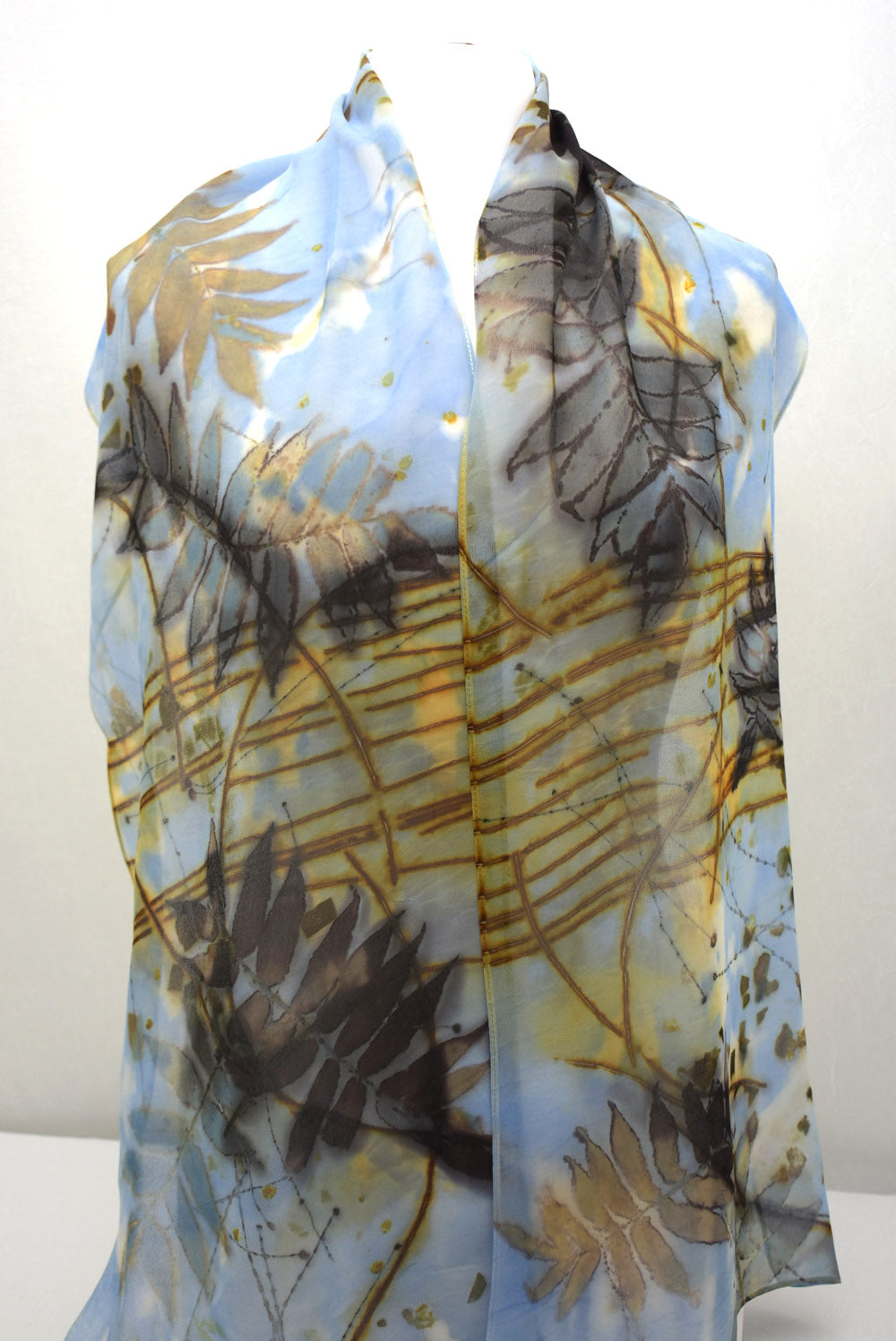This photograph features a sheer blue shawl with an intricate pattern of large leaf and branch designs, gracefully draped around a white torso mannequin. The delicate material allows light to pass through it, enhancing the visual appeal of the botanical motifs. The leaves are depicted in shades of gray with black borders, and brown with darker brown borders. Branch-like brown lines run through the center, adding depth to the design. The mannequin, devoid of head and arms, is mounted on a small stand placed on a flat white surface, likely a table or counter, set against a plain light grey wall. The overall presentation of the shawl on the mannequin highlights its airy, watercolor-like aesthetic and nature-inspired theme.